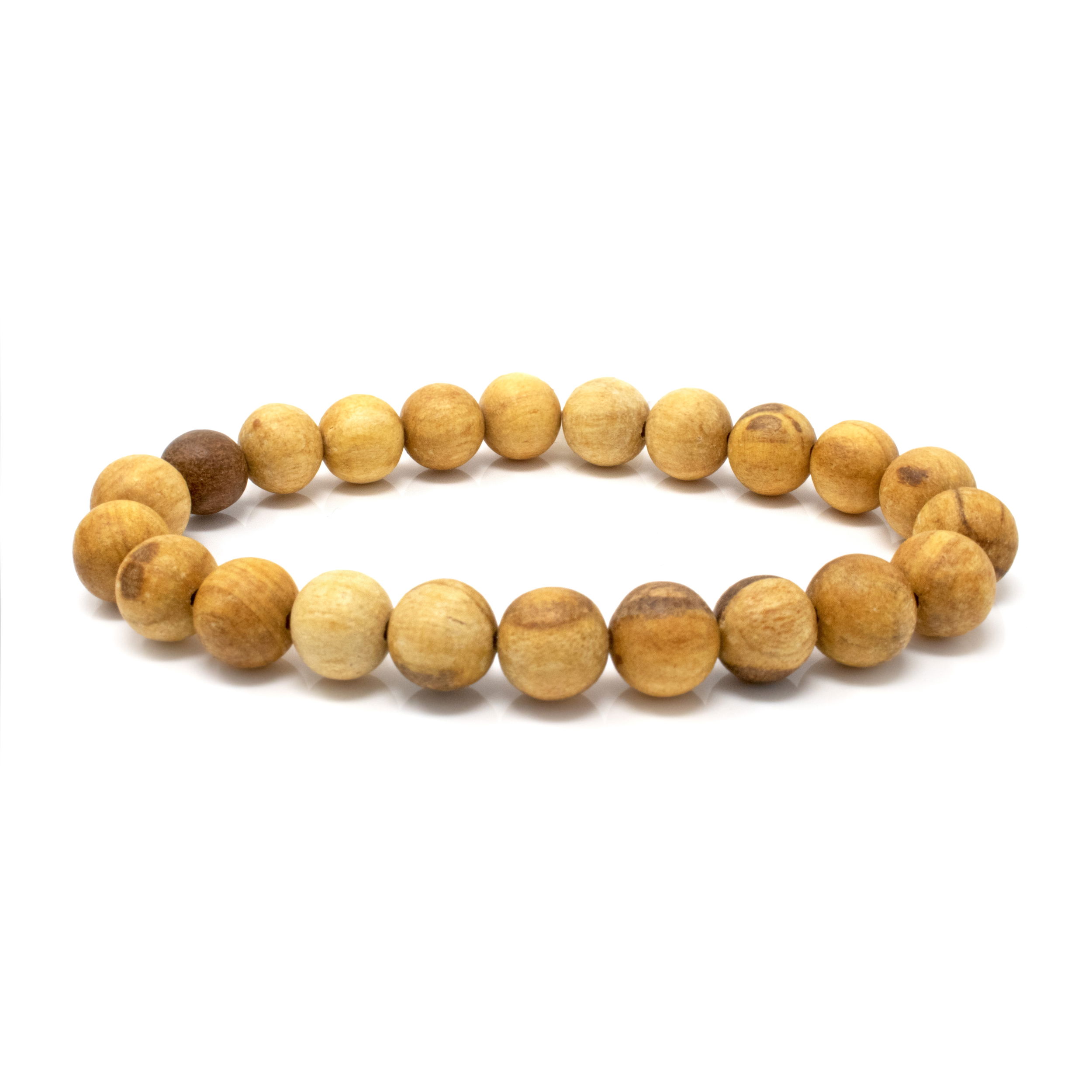The image depicts a beaded bracelet arranged in a circular pattern on a white background. The bracelet consists of medium brown wooden beads, each showcasing unique grain patterns with varying shades of brown, from light to dark. Most of the beads feature different colored streaks and spots, enhancing the natural texture of the wood. Notably, one bead on the left side stands out as a solid dark brown, contrasting with the predominantly medium brown tones of the other beads. These round beads, approximately the size of a dime, cast subtle shadows on the white surface beneath them, indicating even lighting. The bracelet appears to be on an elastic band, with no visible string, suggesting a snug fit as the beads are closely butted against each other. This item, with its earthy aesthetic, might lean more towards being a men's accessory.